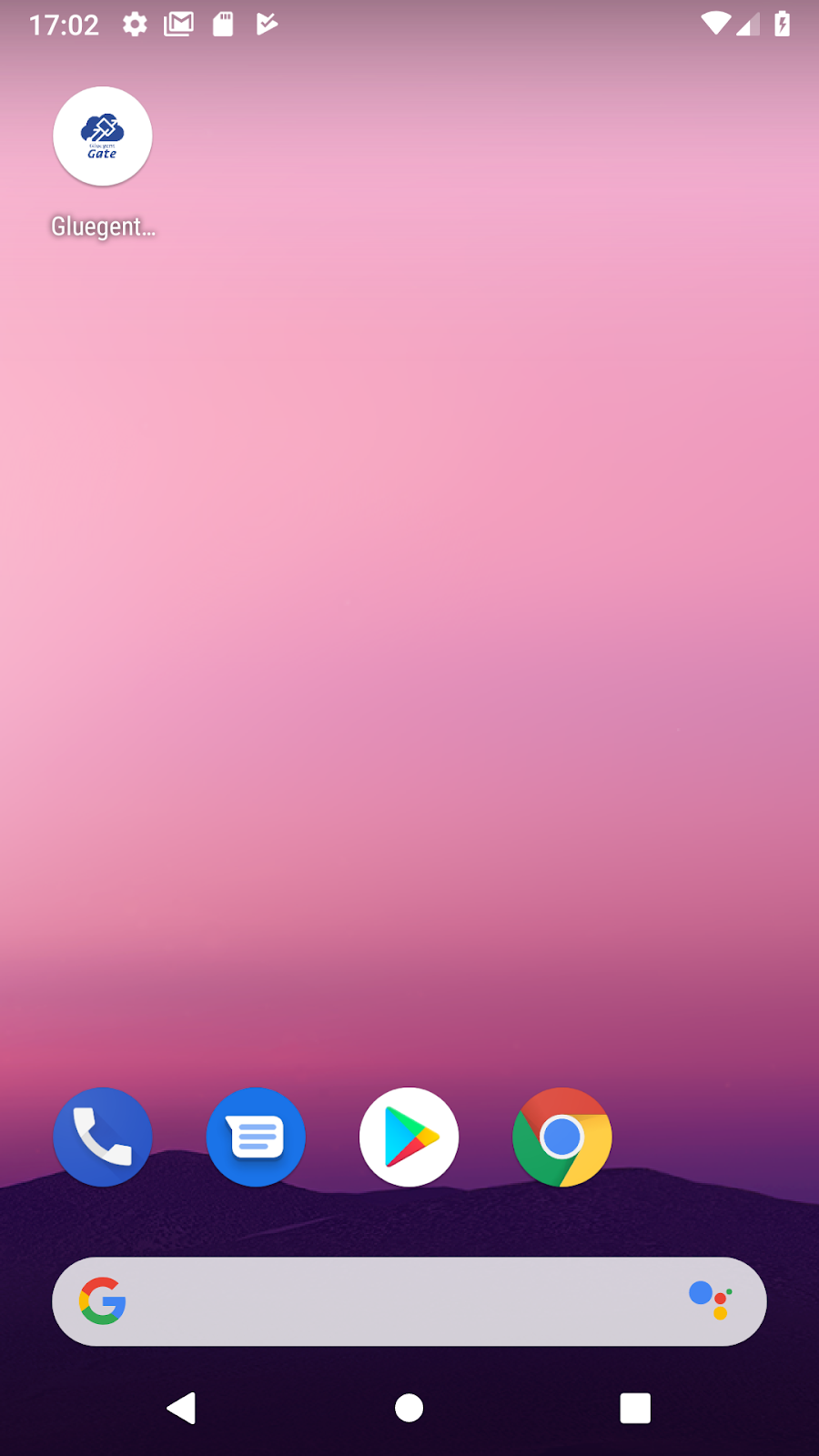The image is a screenshot of someone's cell phone home page. At the top, there is a gradient ombre purple design transitioning to a shadowy, deep purple cliff-like design at the bottom. At the very top, the time is displayed as "1702." Next to the time, there are several icons: a gear symbol, the Gmail icon, an SD card icon, and the Google Play Store icon with a checkmark. On the right side, there are more status icons in white: the Wi-Fi symbol, the mobile data symbol, and the battery symbol.

In the top left corner of the screen is an app icon consisting of a white circle enclosing a blue cloud with indistinct lines on it, accompanied by small text above a larger word that reads "Gate." Beneath this, in white text, it says "gluegent..." Other app icons are aligned at the bottom of the screen. These include a blue circle with a white phone icon for calling, a blue circle with a message blurb box for messaging, a white circle containing the Google Play Store icon, and a multicolored circle that appears to be the Google Chrome icon.

Below these icons, there is a white elongated horizontal oval, featuring a rainbow-colored Google "G" on the left and four colored dots (blue, red, yellow, and green) on the right. 

At the very bottom of the screen, there are three navigation icons: a triangle pointing left, a circle, and a square—all in white. The screen does not contain any additional text.